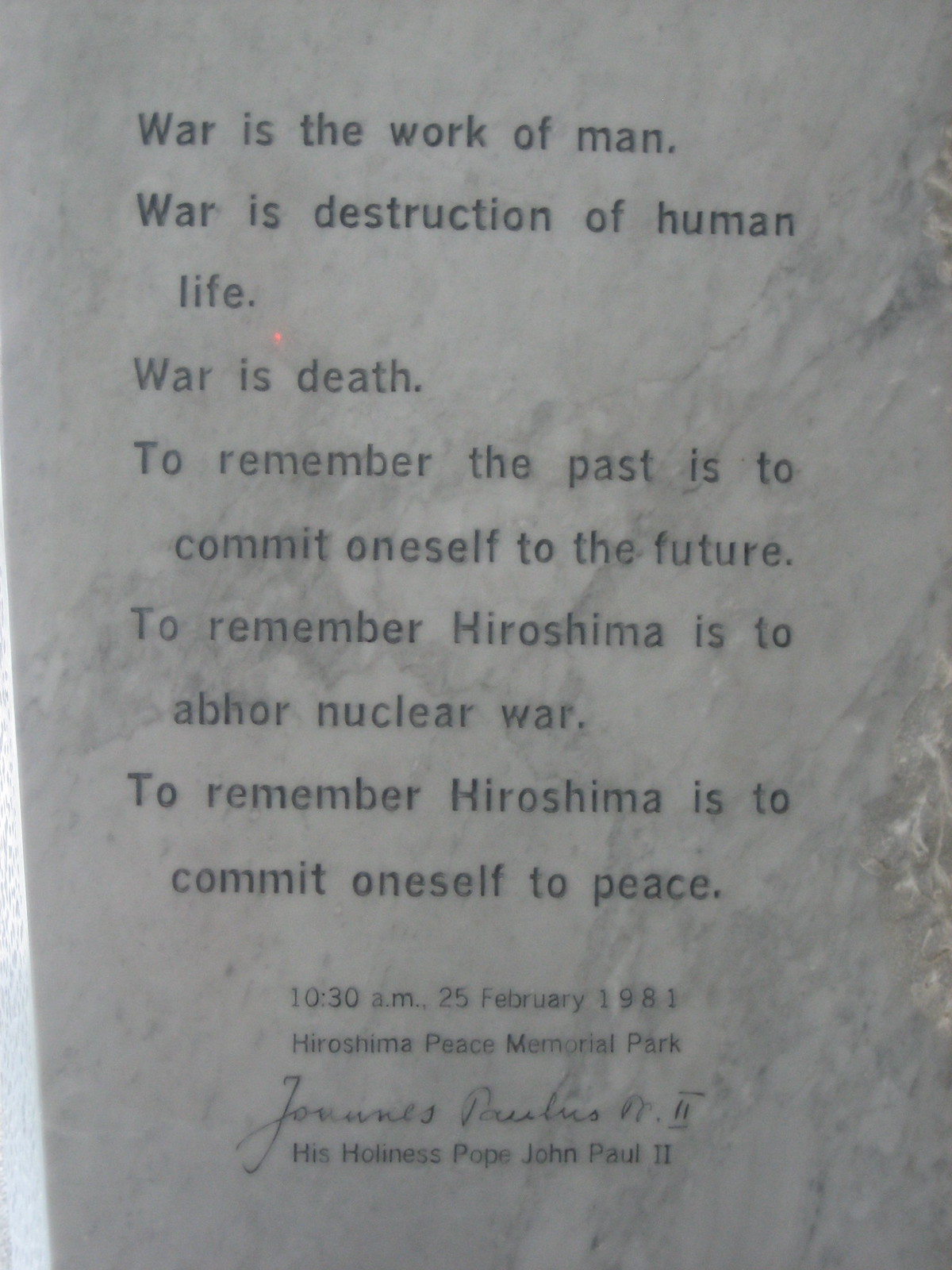This image depicts a close-up of an engraved marble plaque, predominantly grey with a slightly serrated texture. The plaque features a message in black text, conveying a powerful anti-war sentiment. It reads: "War is the work of man. War is destruction of human life. War is death. To remember the past is to commit oneself to the future. To remember Hiroshima is to abhor nuclear war. To remember Hiroshima is to commit oneself to peace." The text is followed by a date and time, "10:30 AM, 25 February 1981," and the location, "Hiroshima Peace Memorial Park." Below this information, the plaque is signed by His Holiness Pope John Paul II, also referred to as Johannes Paulus II.